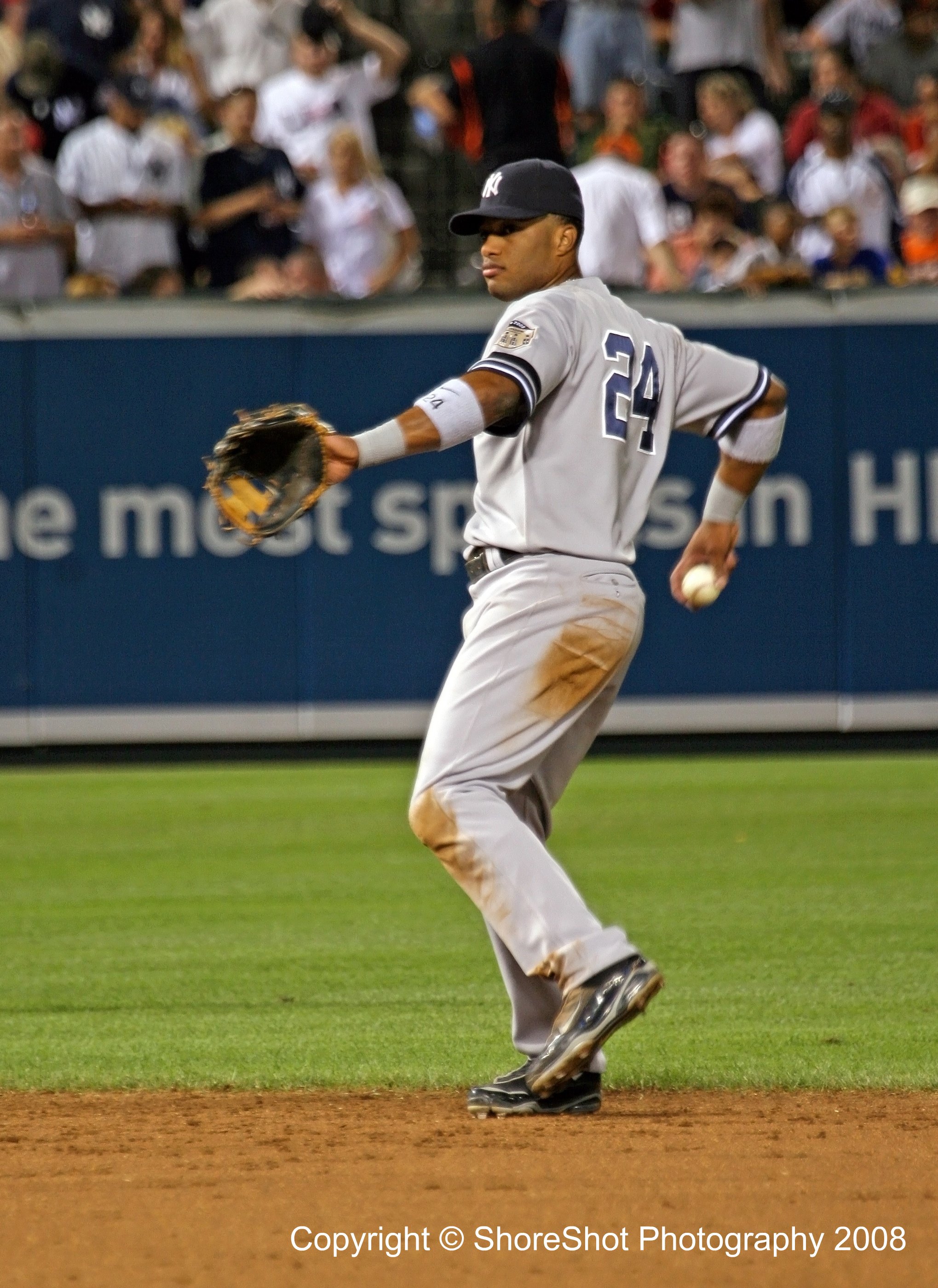This image captures a moment at a baseball stadium, featuring a player in a gray uniform with dark blue lettering and the number 24 on his back. The player, wearing a black Yankees hat with white "NY" text, has visible dirt stains on his pants and knee, suggesting he recently slid. His right hand holds a baseball down at his side, while his glove-covered left hand is ready, his left foot off the ground and knee bent, indicating he is poised to throw. He wears white wristbands and elbow bands. The stadium background features a blue homerun fence and a crowd of fans, many dressed in jerseys, conversing and eating. The copyright "See Sure Shot Photography 2008" is noted in the image. The scene blends the green grass of the outfield with the infield dirt where the player stands.